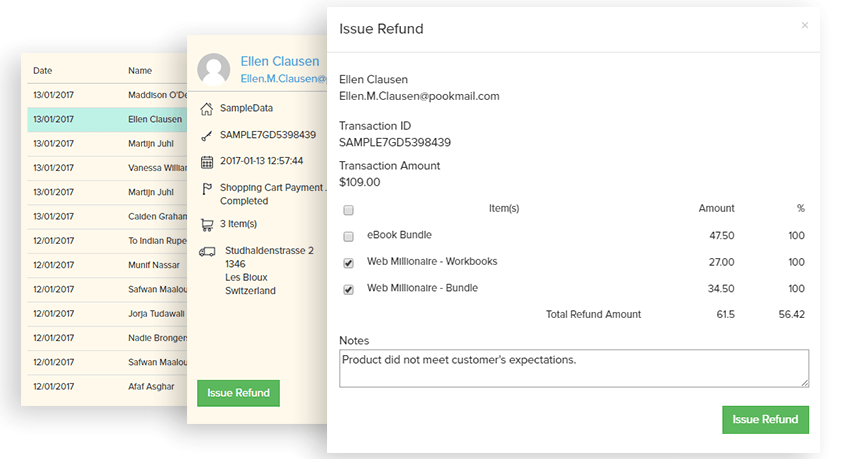The image depicts a stacked arrangement of three digital screenshots, with the prominent one on the top right detailing an issue refund page. At the top of this screenshot, it reads "Issue Refund," followed by customer information: Ellen Clausen with the email ellenmclausen@pookmail.com. The transaction ID is given as SAMPLE7GD5398439, with a transaction amount of $109.

The transaction breakdown lists:
- **eBook Bundle**: $47.50 with a discount percentage of 100%.
- **Web Millionaire Workbooks**: $27 with a discount percentage of 100% (noted with a checkmark).
- **Web Millionaire Bundle**: $34.50 with a discount percentage of 100% (also noted with a checkmark).

A note at the bottom states: "Product did not meet the customer's expectations." A green "Issue Refund" button is prominently located at the bottom of the page.

The second screenshot, partially visible in the middle, seems to provide various views of the customer’s order details and cart contents, likely showing more specific contact information and another green "Issue Refund" button.

The third screenshot, faintly discernible in the background, appears to display a list of all orders related to the products, with visible columns mainly including dates and customer names.